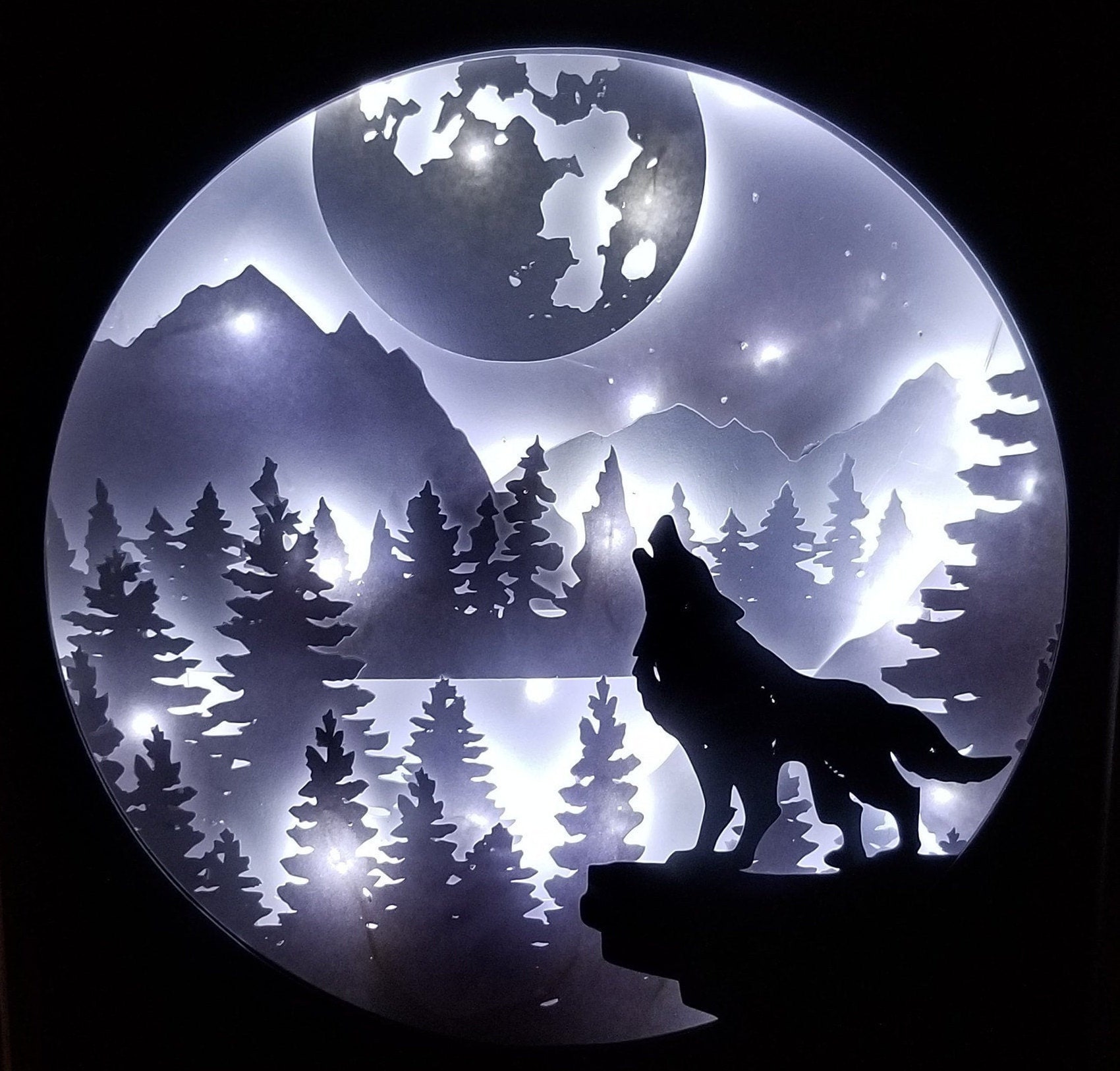The image is a meticulously crafted metal artwork centered in a square with a black background. Dominating the composition is a large, round circle positioned centrally but slightly above the horizontal midpoint. This circle contains a vividly detailed landscape rendered in various shades of gray and silver. At the top left of this circle, there's a darker-colored moon or planet, partially visible, with silver highlights marking its craters and land masses. Meanwhile, the background within the circle features a subtly shimmering gray sky dotted with sparkles, suggesting a starry night.

Descending from the sky, the art reveals a series of mountains in varying hues of gray—one notably darker on the left with an illuminated peak, and lighter ones extending to the right. Below the mountains lies a tranquil lake, its surface depicted in light gray, flanked by clusters of silver evergreen trees scattered across the midsection and lower parts of the circle. These trees frame the reflective water, adding layers of depth to the scene.

Anchoring the scene at the bottom right of the circle, set against the encompassing black backdrop, is an intricate silhouette of a wolf perched on a rocky ledge. The wolf, rendered in stark black, faces left with its head tilted upward, appearing to howl at the larger circle, which symbolizes the moon. This multi-layered metal art elegantly combines natural elements within the circular frame, creating a striking contrast against the dark background and emphasizing the serene, yet wild beauty of nature.